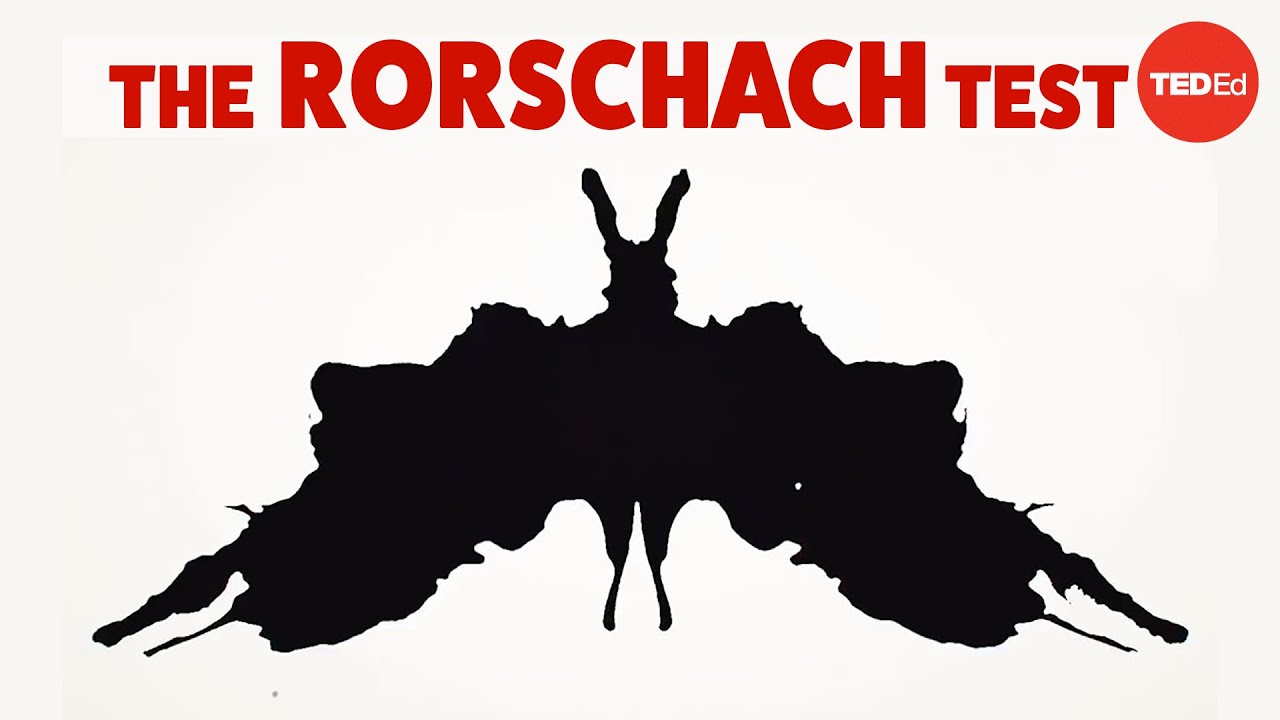The image appears to be a poster for a TED Talk event, set against an off-white background. Dominating the top portion of the poster in bold, dark red lettering are the words "The Rorschach Test." To the right of this title is a circular red orb containing the white text "TED-ED." Beneath the title, there is a large black inkblot, centrally placed, resembling a traditional Rorschach test image. The inkblot features symmetrical shapes that could be interpreted as a moth or bat, with distinguishable antennae-like projections and expansive wings stretching to either side. The body of the inkblot appears to have two black lines hanging down, further suggesting the legs or feet of the depicted insect-like figure.